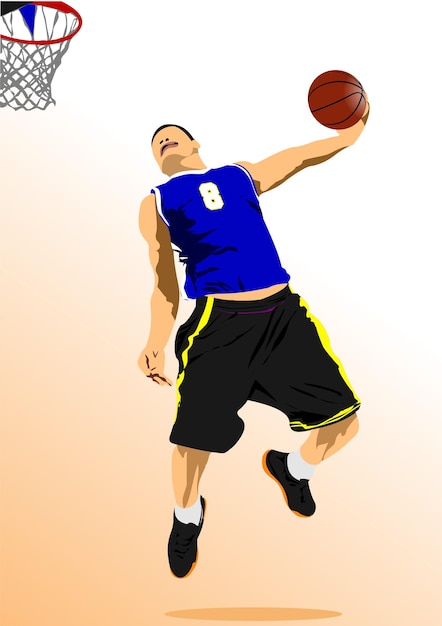The image is a detailed piece of digital vector art depicting a basketball scene. The background features a gradient transitioning from white in the upper right to a peachy-orange hue in the lower left. In the upper left corner, a red basketball hoop with gray netting is prominently visible. A white basketball player is captured in mid-air, seemingly about to dunk a brown basketball with black lines, held in his right hand. The player has short black hair and is dressed in a blue sleeveless athletic shirt with a white number 8 on it. He sports black pants with yellow stripes down the sides and black athletic shoes with orange soles, complemented by white socks. The artwork includes some detailed elements, such as the attire and the basketball, but the player's hands and face are less refined, with peculiar features like no eyes and an odd-looking mouth. Overall, the scene conveys dynamic action despite the cartoony and somewhat simplistic rendering of the character.